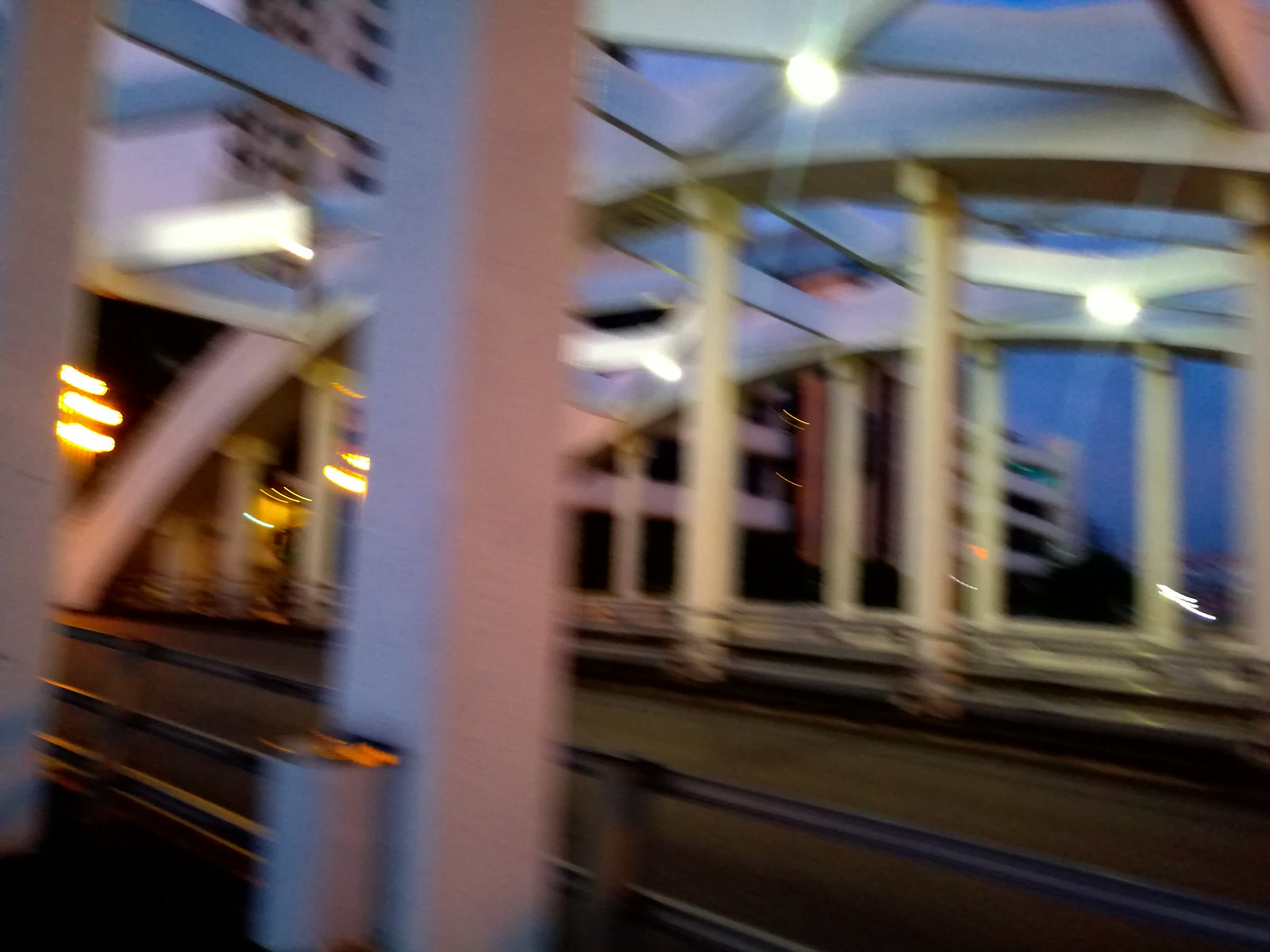Blurry evening shot focusing on an architectural structure that appears to be a bridge, characterized by pinkish-bronze pillars and a metal frame resembling a fence. Beyond the bridge, tall buildings loom, enhancing the urban backdrop. The bridge's interior, partially visible through the hazy image, showcases a series of supporting columns and a metal pipe-like fence that runs diagonally from the bottom right to the bottom left, contributing to the industrial aesthetic of the scene.